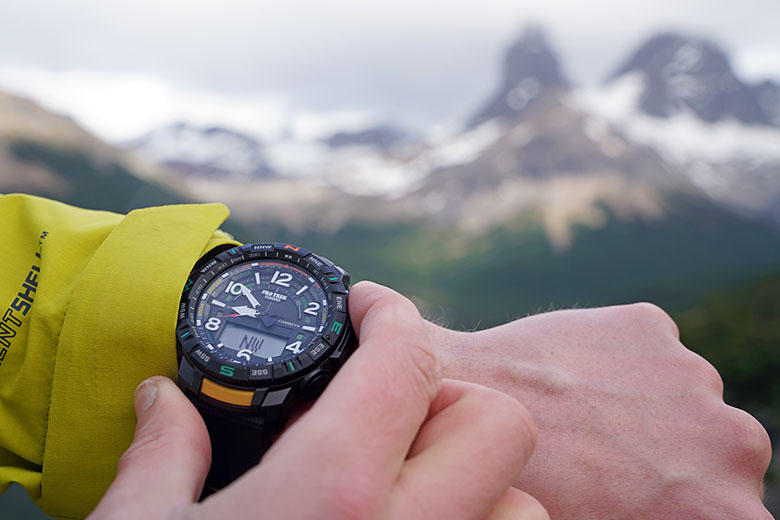In this detailed, color photograph, the main focus is on a large black sports watch with prominent white numerals at 12, 2, 4, 6, 8, and 10, and a small rectangular digital screen displaying "NW" for the direction. The watch is being worn on the pale white wrist of a man, whose left hand is seen adjusting the dowel or buttons on the watch, possibly setting or checking the time, which reads 10 till 9. The man is dressed in a yellow raincoat, part of whose sleeve is visible. The background is artistically blurred, revealing a snow-capped mountain range with a green forest at its base. The out-of-focus mountains and nature scene add depth to the image, contrasting with the sharply focused watch and hands.